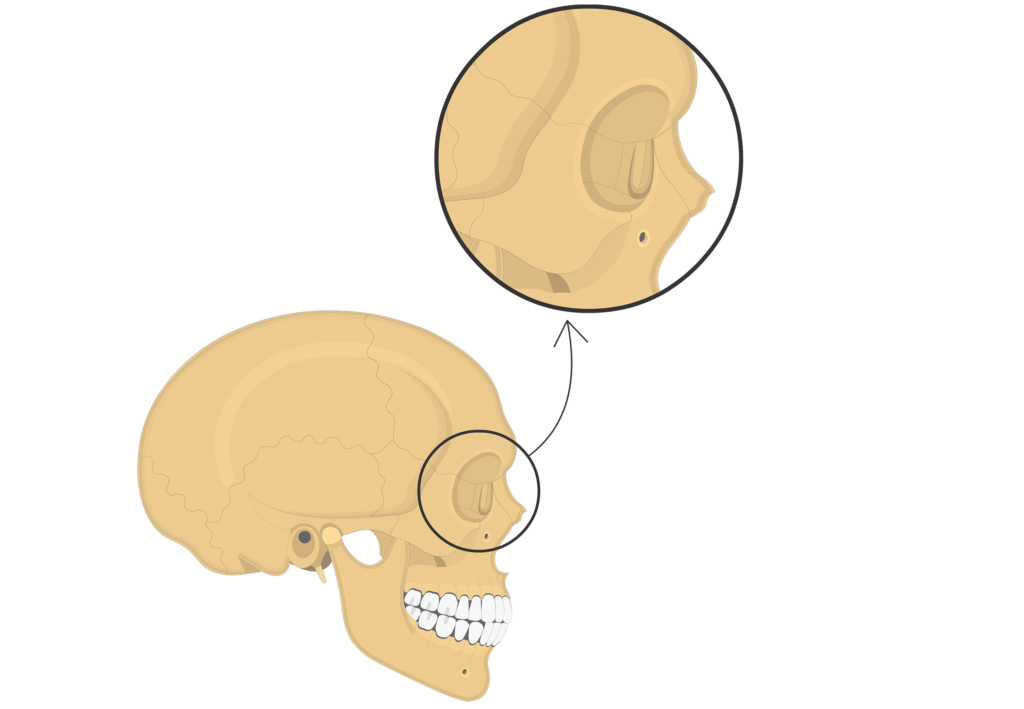This detailed illustration depicts a tan-colored human skull shown in profile, facing left. The skull, rendered with minimal detail, features a complete set of teeth and includes a few faint lines indicating cracks, particularly near the ear extending toward the back and top. A thin black circle is drawn around the eye socket, cutting into the nose area, with an arrow pointing from this circle towards the top right, where it connects to a larger black circle displaying a close-up view of the eye socket. Additionally, there are two small holes in the skull—one located under the eye socket and another on the jawline. These detailing elements aim to highlight specific anatomical structures, though the purpose of the holes is not immediately clear.